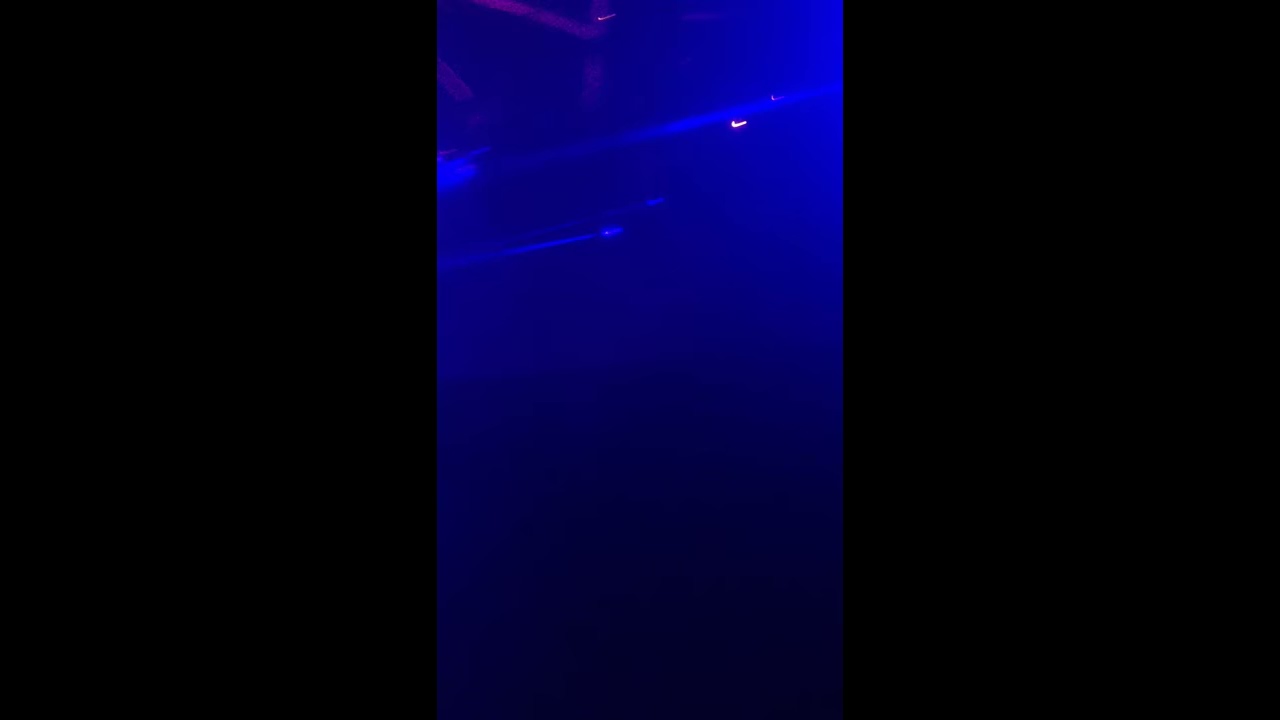This image is very dark, divided into three equal sections with the right and left sections completely black. The central portion is a dark blue that fades into the blackness at the bottom. The top part of this central section features a few thin, lighter blue lines and a tiny white line, giving the appearance that it might be underwater, with a couple of small red dots at the top. The blue color lightens as it moves upwards, resembling a royal blue hue. The central panel also shows three darker blue streaks running horizontally from left to right. The bottom streak is the thickest and stops halfway through the image, the middle streak extends slightly further to the right, and the top streak spans the full width of the central section. No text or words are present in the image. The overall effect suggests a dark room with blue lights, potentially evoking the ambiance of a concert or a similar event.